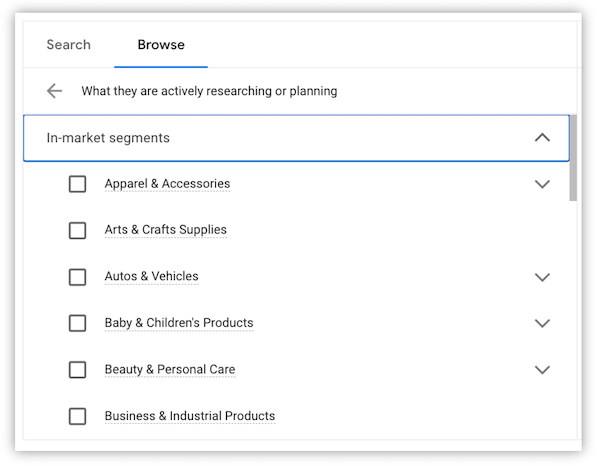The image depicts a user interface layout for a market research platform. In the upper left corner, the word "Search" is displayed in gray. Adjacent to it, the word "Browse" is written in black text and underlined in blue, indicating it is the currently selected option.

Below this text, there is a left-arrow icon followed by text that denotes what the user is actively researching or planning. Underneath this section, there is a long rectangular box outlined in blue containing the text "In Market Segments" and featuring an upward-pointing arrow.

Beneath this rectangle, there are six squares arranged in two rows. Each square is associated with a label to its right. 

- The first, smaller square is beside the label "Apparel and Accessories."
- The second square is beside "Arts and Crafts Supplies."
- The third square is beside "Auto and Vehicles."
- The fourth square is beside "Baby and Children's Products."
- The fifth square is beside "Beauty and Personal Care."
- The sixth square is beside "Business and Industrial Products."

Each label corresponds to a category within the market segmentation being displayed.